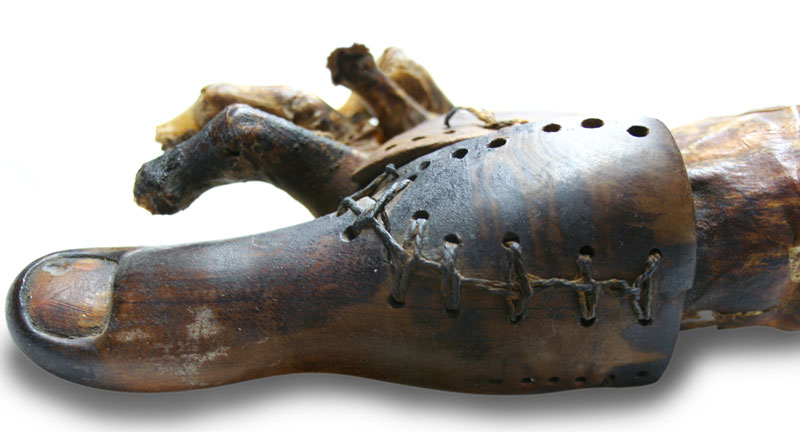This image shows a close-up of an ancient, possibly archaeological artifact that appears to replicate a human right foot and part of the lower leg. The foot is crafted from a dark material with a wood-like texture, potentially wood itself, and displays significant signs of aging, including darkening and areas of wear and deterioration. Detailed contours faithfully mimic the natural shape of a human foot, exhibiting individually defined toes. The big toe is particularly notable for its detailed craftsmanship, including a lighter, tannish brown coloration where the nail would be. The second toe is bent and darker, while the subsequent toes show varying degrees of decay, with some appearing skeletal or amputated. 

A series of holes are drilled into the foot, beginning near the toes and extending along the top. This area features evidence of repair, with a section stitched together using what appears to be a leather strip, reminiscent of shoelaces or old baseball glove lacing. The artifact evokes an eerie sensation as some toes resemble bare bones, hinting at a blend of organic and artificial materials. This composition suggests it might be a prosthetic or substitute limb, crafted to replace a missing appendage, and intriguingly combines elements of both wood and bone, reflecting its ancient origin and the reverence for utilitarian craftsmanship of the past.